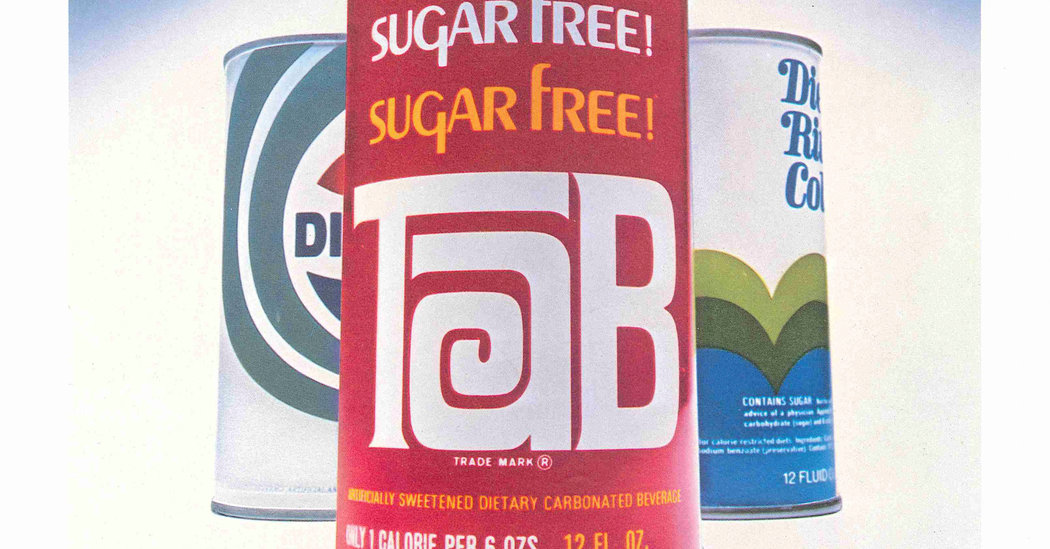This image showcases three vintage cans of Diet Cola prominently displayed. 

1. **Center Can: Tab**
   - The focal point of the image is a pink can of Tab. The can features bold, white letters proclaiming "Sugar-Free!" at the top, with a second declaration in orange letters just below. Dominating the center of the can is the iconic "Tab" logo with its distinctive spiraling "A". Beneath the logo, the term "Trademark" is clearly marked, followed by the phrase "Artificially Sweetened Dietary Carbonated Beverage," which emphasizes the low-calorie content. The can specifies that it contains only one calorie per six ounces, and the total volume is 12 fluid ounces.

2. **Right Can: Diet Rite Cola**
   - To the right, a can of Diet Rite Cola is turned slightly away, offering a partial view of its label. The text "Contains sugar" is somewhat visible, hinting at its distinctive formula. The can's design combines a primarily white background with striking green and blue sections, adding a dynamic visual contrast.

3. **Left Can: Diet Pepsi**
   - On the left side of the image, there is a partially visible can of what appears to be Diet Pepsi, identified by its familiar color scheme. Despite only a fragment being visible, the recognizable design elements suggest it's another classic diet soda option.

Each can represents a unique piece of soft drink history, showcasing the varied branding and marketing strategies of diet colas from a bygone era.